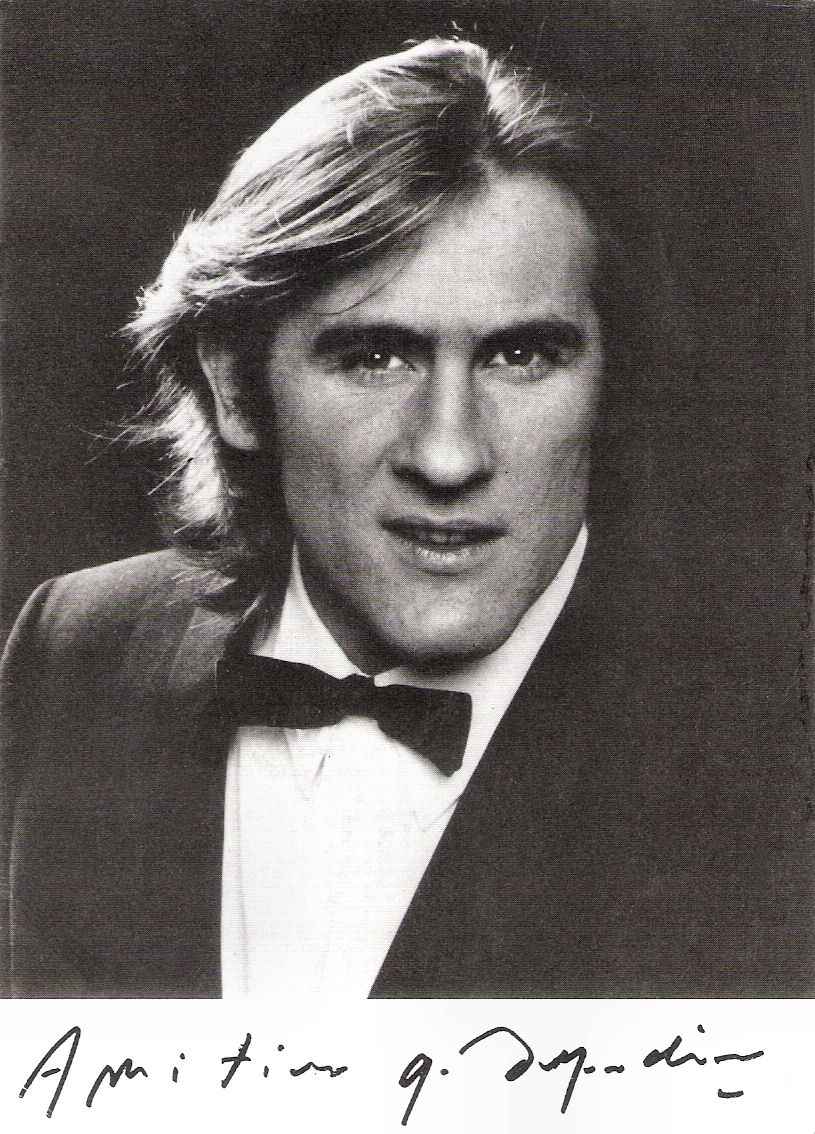This black-and-white promotional photo features a man with light skin and shoulder-length, flowing brown hair, dressed in a tuxedo with a black jacket, white shirt, and black bow tie. He is looking directly at the camera with a half smile against a plain black background. At the bottom of the image, there is an illegible signature, possibly written in black ink, that appears to start with "A-M-I-T-I" followed by an indistinct middle initial and a difficult-to-decipher last name.